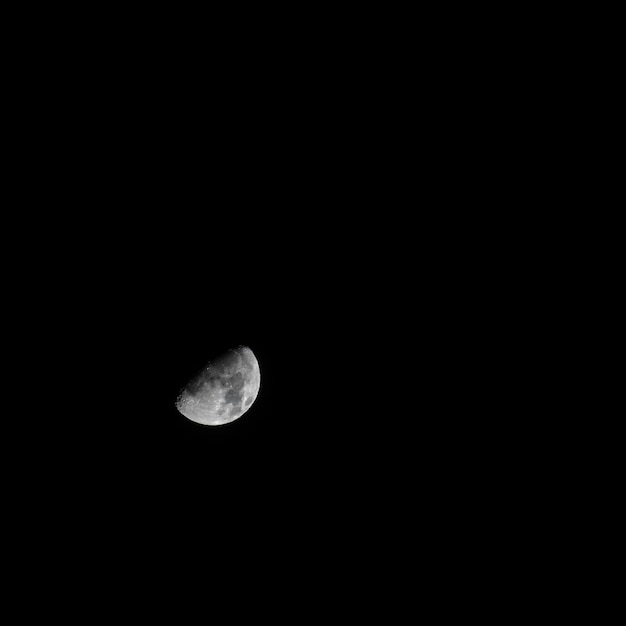The image is a monochromatic photograph capturing part of the moon against a pitch-black night sky. No stars or clouds are visible, leaving the background completely black. The moon is small in the frame, with only about two-thirds of its surface showing, primarily the lower right portion. This section of the moon features various darker gray spots and craters typical of lunar landscapes. The subtle variations in gray tones highlight the textured surface of the moon, creating a striking yet simple composition.